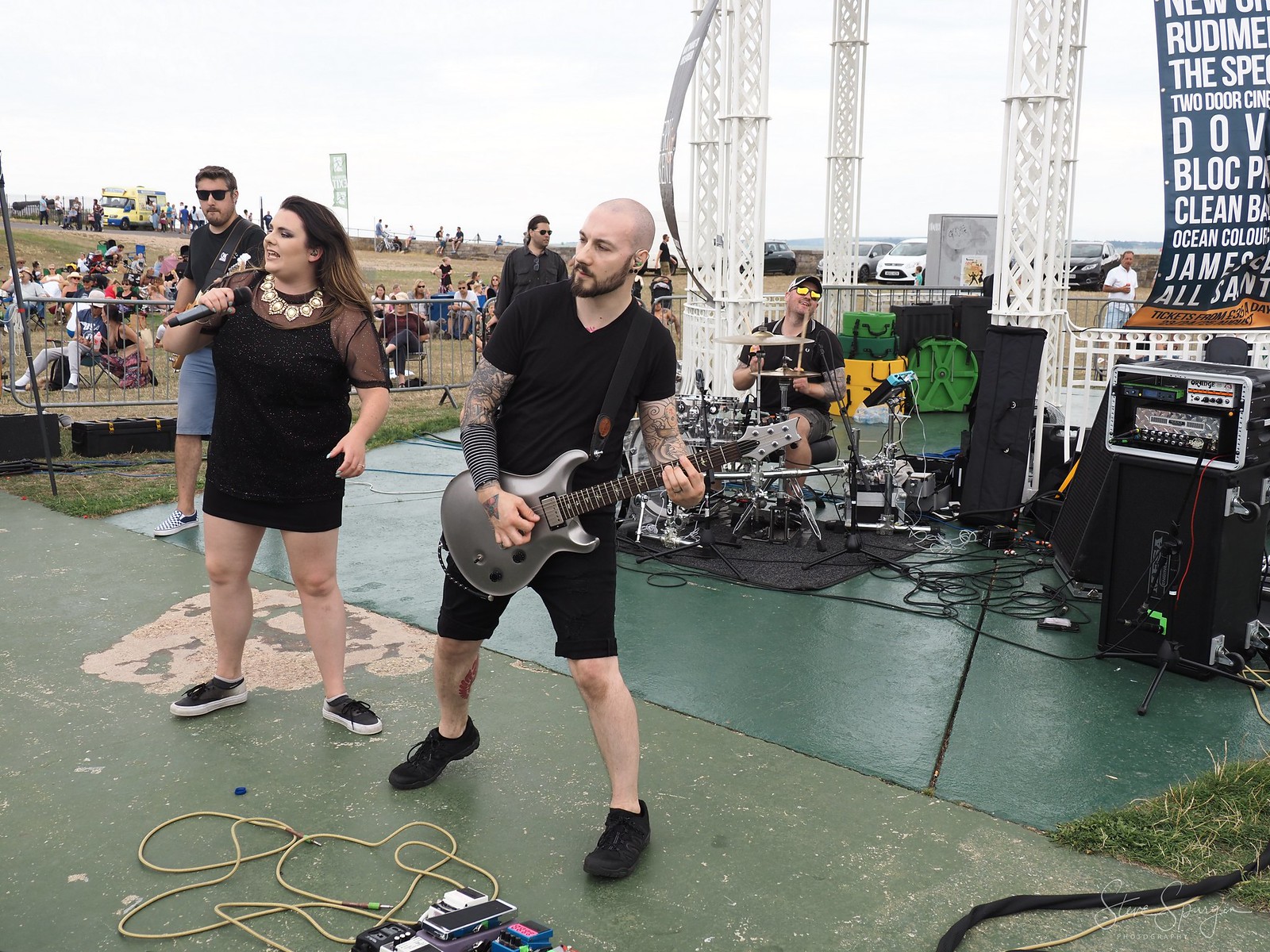In this outdoor concert setup, three performers are on stage against a backdrop of white clouds and patches of blue sky, with a crowd seated in a grassy field behind them. Center stage is a well-built woman with tennis shoes who is singing into a microphone. She wears a strikingly short, black dress that falls just above her knees, complemented by a very large necklace. Partially obscured behind her is another individual. To her right stands a man in all black attire, featuring shorts, a shirt, and matching tennis shoes. His arms are covered in tattoos as he plays his guitar. Behind them, perched on a black carpet, is a drummer wearing sunglasses, a hat, a short-sleeved shirt, and shorts, also adorned with tattoos. The stage is subtly detailed with yellow wires and effects pedals scattered around, adding to the vibrant energy of the scene.